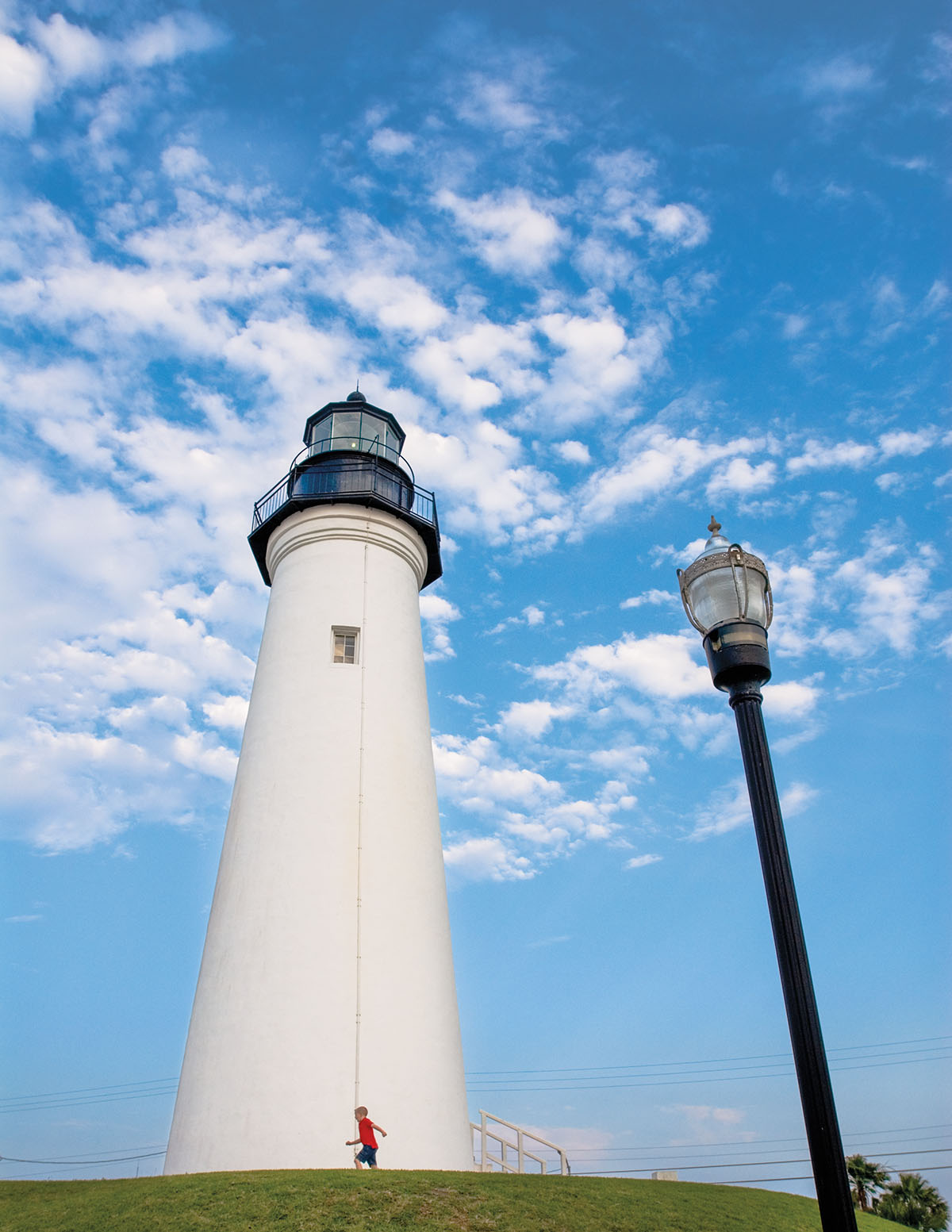A vivid image captures a serene scene dominated by a vast blue sky filled with puffy white clouds that extend down three-fourths of the picture. The foreground features a verdant grassy hill, viewed from a lower perspective, giving the viewer a sense of looking upwards. At the top of this hill stands a prominent white lighthouse, complete with a black railing at the top and a window below it. The lighthouse extends slightly above the middle of the image, with its wider lower level tapering to a narrower upper section. Centrally placed in the lower part of the image, a young boy wearing blue shorts and a red shirt sprints sideways towards the left. Additional details include a dark metal light post situated in the lower right corner and spindly telephone wires running across the lower portion of the scene. Together, these elements create a picturesque and dynamic composition.